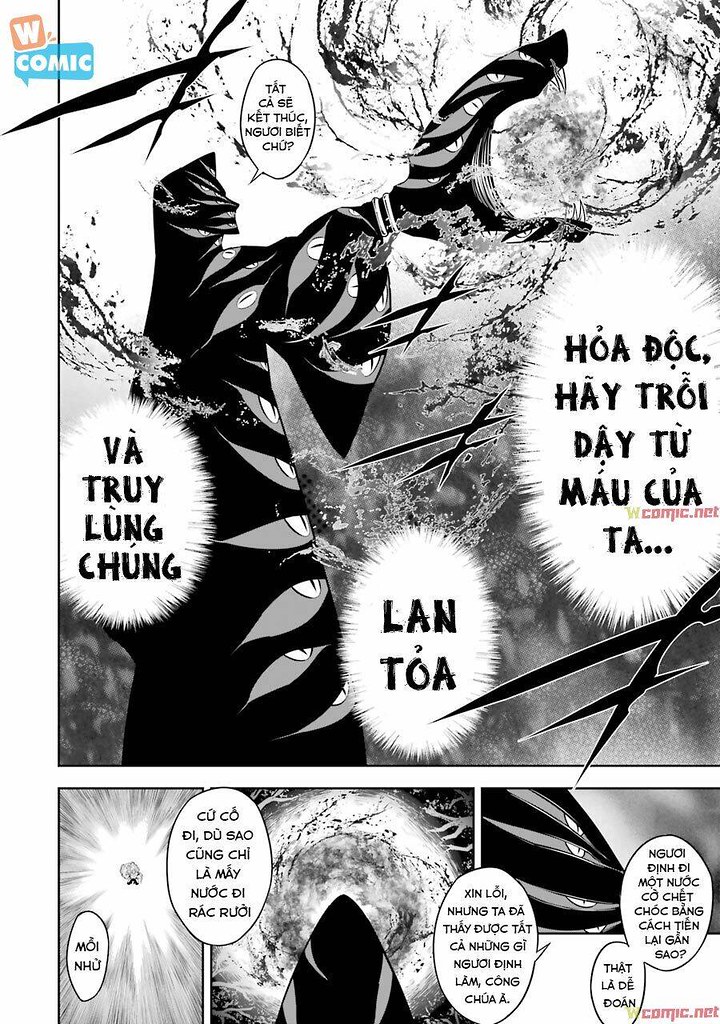The image is a detailed black and white page from a comic book, possibly a manga, prominently featuring a surreal, human-shaped creature covered in multiple snake-like eyeballs. The creature's hand, also shaped like a snake's head and covered in eyes, appears to be channeling a fireball. The comic page includes several speech bubbles filled with an Asian language, likely Vietnamese. There are minimal colors in the otherwise monochrome image, with hints of orange, light blue, white, black, various shades of gray, pink, and olive green. The top left corner displays a logo reading "W Comic" within an orange square, accompanied by a speech bubble with the word “comic” inside. The bottom of the page features the site name “W Comic dot net.”